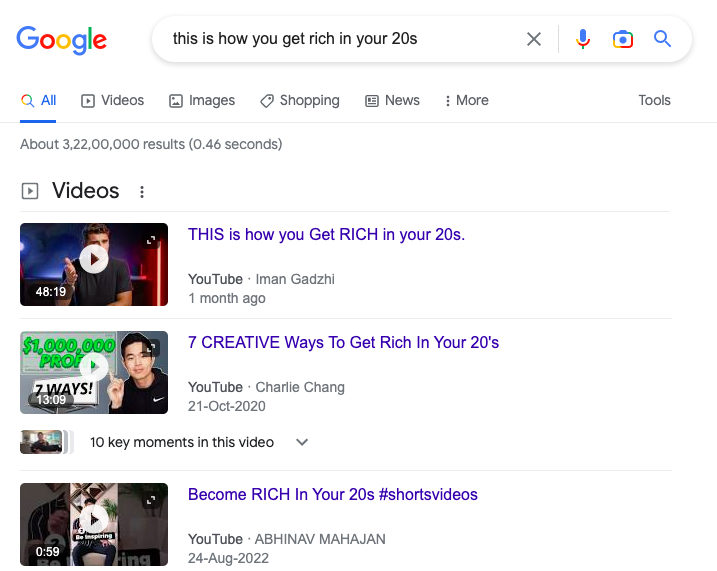The image is a screenshot of Google search results. In the top left corner, the colorful Google logo, displaying the word "Google" in blue, red, yellow, blue, green, and red, is prominently visible. Below the logo is the capsule-shaped search bar, within which the user has typed, "how to get rich in your 20s." To the right of the search text are icons for deleting the search (an 'X'), voice search (a microphone), image search (a camera), and initiating the search (a magnifying glass).

Beneath the search bar, a navigation menu offers various search categories: "All," "Videos," "Images," "Shopping," "News," and "More" options, with "Tools" located on the far right. The "All" tab is currently selected, showing a result count of approximately 32,200,000, which were delivered in 0.46 seconds.

The top three search results displayed are all videos from YouTube. The first video, titled "This is how you get rich in your 20s," has a duration of 48 minutes and 19 seconds. The second video, "7 creative ways to get rich in your 20s," is 13 minutes and 9 seconds long and comes with an option to view 10 key moments from the video. The third video, labeled "#shorts," is a brief 59-second clip titled "Become rich in your 20s."